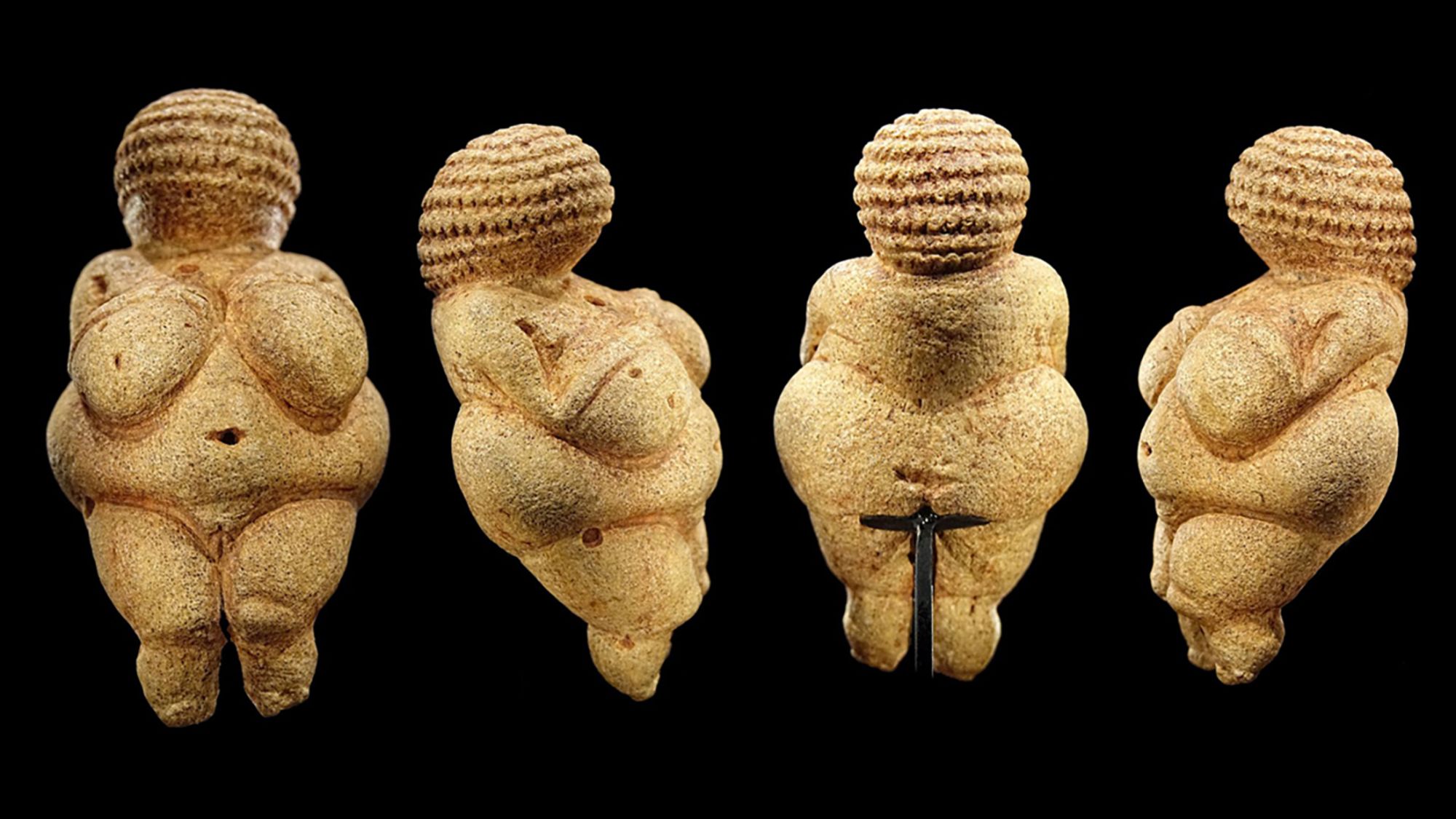The photograph showcases a small, highly stylized statuette depicted from four different angles within a rectangular frame, against a black background. The statuette, appearing to represent an overly exaggerated, overweight naked woman, possesses prominent physical features: thick, short legs; a round, oval-shaped body; and large breasts. Her arms are crossed and rest on her chest, and her navel is indicated by a small pit on her stomach. The head is adorned with curved lines that likely signify hair or braids, though there are no discernable facial features. The four angles include a front, right side, back, and left side view, meticulously edited to appear as one comprehensive image. The sculpture, detailed with minute carvings and seeming to be hand-crafted, may evoke the art of an ancient civilization, reminiscent of caricatured human forms. Despite its exaggerated proportions, the statuette is small enough to fit in the palm of a hand. The intricate details and multiple perspectives highlight the craftsmanship and artistic intention behind this unique artifact.